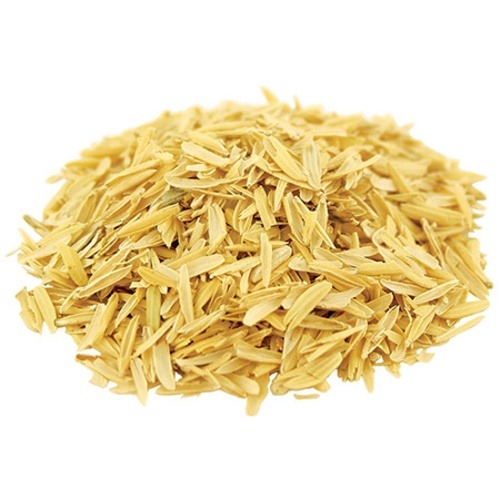This image showcases a substantial pile of grain-like material, possibly wheat or rice husks, resting on a completely white background. The pile, about four inches tall and the size of a handful, consists of flattened, pale yellow pieces with occasional hints of brown and green. The texture appears dried, suggesting it could be grain husks or a type of pasta cut into smaller, thinner pieces resembling seeds or flattened rice. The arrangement of countless varieties of these small seeds or husks gives the impression of a harvest, gleaming with an overall yellow tone but interspersed with subtle variations in color.